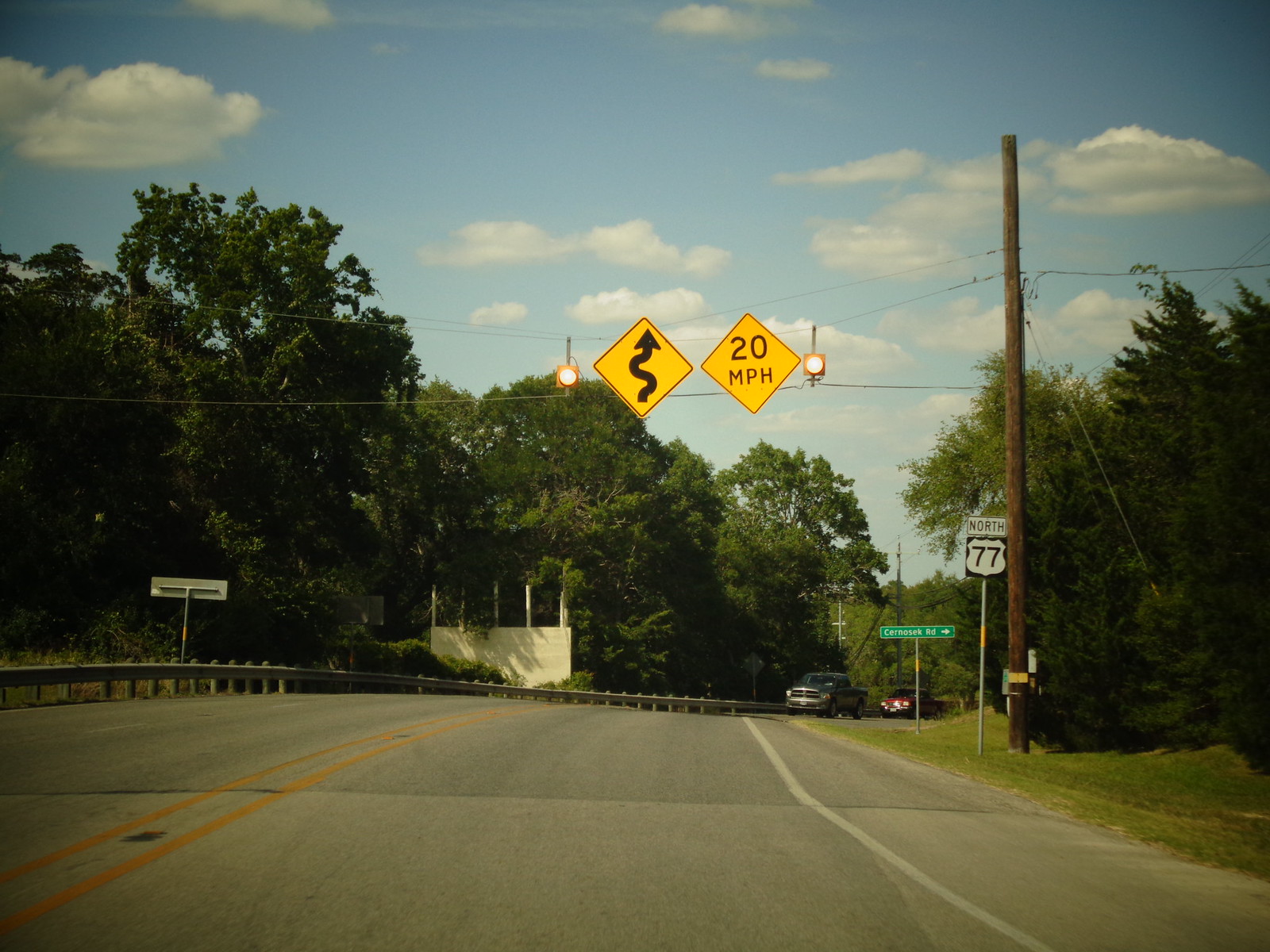This landscape photograph features a vivid scene with a striking blue sky dotted by sparse white clouds stretching from the upper left to the upper right corner. Dominating the lower half, the road's dark macadam extends from the lower left to the lower right corner of the image.

In the left center of the photograph, a lush canopy of green tree leaves extends horizontally towards the right center, gradually thinning out where the road ascends and curves. Emerging from this road are several vehicles, notably a blue truck in the lead followed by a red truck.

Flanking these vehicles, a green sign indicating "CERNOSEK Road" is prominently positioned, alongside a Route 77 North sign to its right. Further to the right stands a large telephone pole, adorned with a small yellow and white sign at its base. The pole hosts several wires: one descends to anchor it to the ground, while others stretch across the road to the left.

Suspended along these wires are two lights, illuminating two yellow warning signs below. On the left, a sign indicates a highly winding road ahead, while a sign on the right advises a speed limit of 20 miles per hour.